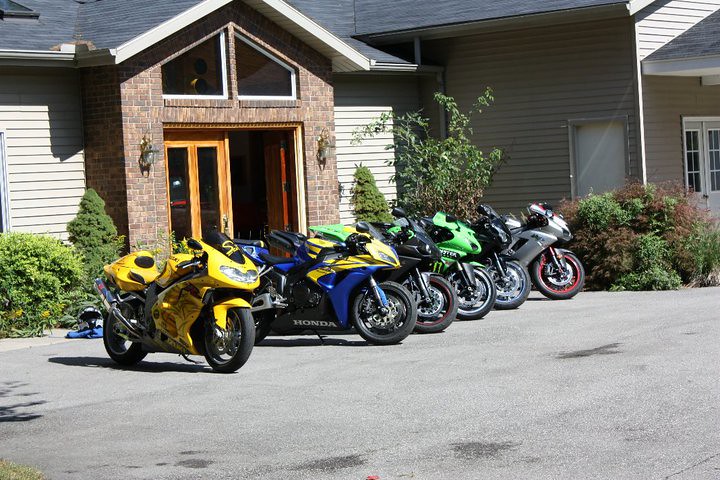This is a detailed outdoor color photograph taken on a bright day. The main focus of the image is a collection of six new, sporty motorcycles parked in a row on an asphalt parking lot. The motorcycles are positioned front-facing the viewer, idenitified by their colors: yellow, blue with yellow detailing, black, green, another black bike, and silver. The bikes are designed for speed with handles tucked behind windshields. 

In the background, there is a single-story building that appears to be an office. The building features a brick entryway with brick columns and a triangular divided window above. The double wooden doors at the entrance have glass panes, with the right door open and the left one closed. Adjacent to the doors, large downward-facing sconce lamps are mounted on the brick columns. The rest of the building is covered in tan horizontal siding, likely vinyl or clapboard, and it has a gray shingle roof where a solar panel is visible in the top left corner.

The area around the building is landscaped with evergreen and conifer shrubs, and additional lower shrubs. In the right background, there’s an L-shaped extension of the same building, featuring tan siding and casting a slight shadow. The right section of this structure also has white rectangular windows and a door. No text or additional elements are present in the image, maintaining a sharp focus throughout.